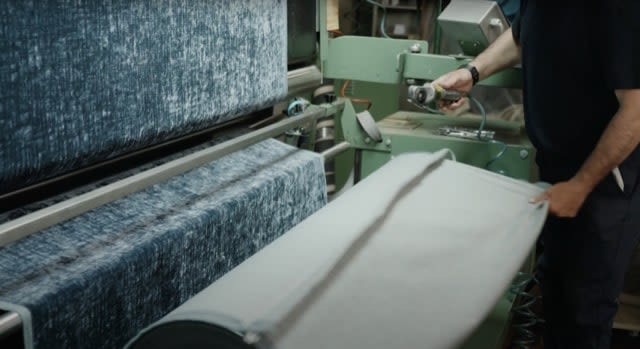The image depicts a factory worker operating a textile mill machine. On the left side, a roll of fabric—bluish with horizontal and vertical patterns against a white background—feeds into the machine, passing under metallic bars and emerging on the floor. The worker, dressed in black slacks, a short-sleeve black top, and a black watch on his right wrist, holds the cloth with his left hand and wields a cutting tool in his right hand. The fabric appears to loop over to the right side of the machine, where the worker is stationed. Behind the worker are various green-colored machines and instrumentation, though their specific functions are unclear. The cloth's appearance suggests a possible blue velvet texture.